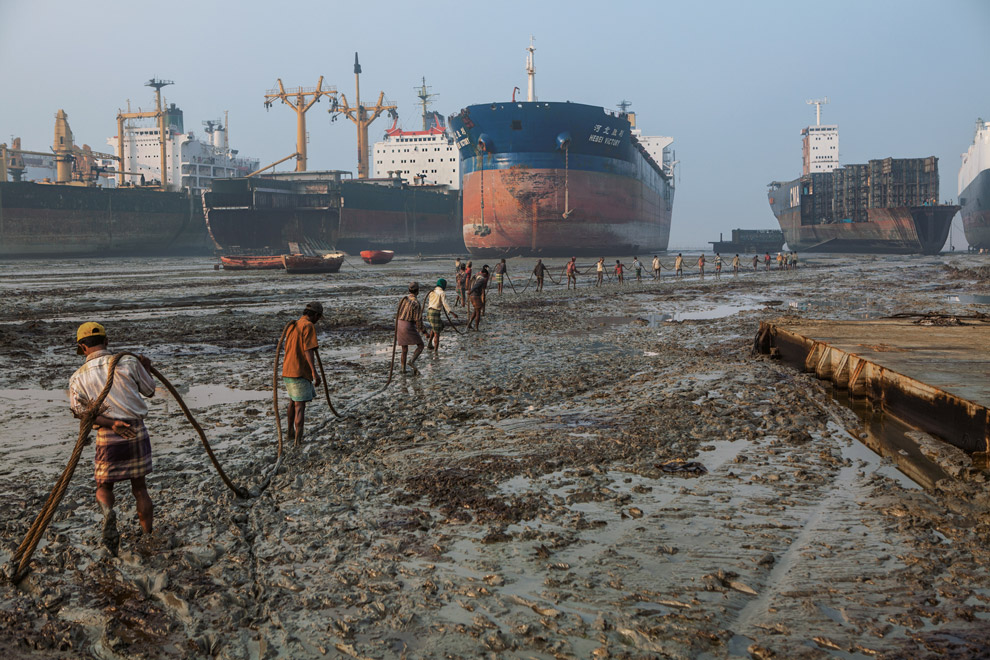This is a real-life photo of a laborious scene set in a muddy, waterlogged boatyard. The foreground features a long line of people, most in shorts and shirts, some wearing baseball caps, hauling what appears to be a heavy hose, though it could also be a rope. They are situated in murky, thick, brown water, stretching from the left side of the image toward one of several large, partially submerged ships. To their right rests a hollow, square-shaped black and brown object on the muddy ground.

The background showcases various large ships. On the top right, there is a black and brown ship with a slender, white structure on top. Centrally positioned, the largest ship boasts a red bottom and blue top with two anchors at its front. Next to it, on the left, another ship features two prominent orange metal projections and a white superstructure. Further left, another vessel displays a large white superstructure with several sizable yellow protrusions. The surrounding area contains scattered smaller boats and possible pier or dock elements on the right, adding to the scene of industrial maritime activity. The overall atmosphere is one of hard labor in a gritty environment, likely in a foreign setting.